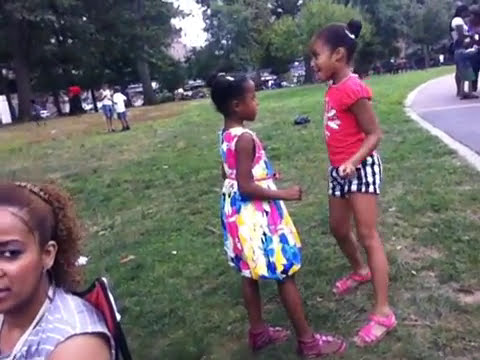In this detailed photograph, set on a sunny summer day in an outdoor garden or public park, the scene is brimming with activity and life. The garden is covered with lush green grass and features a curved, paved footpath on the right, bordered by a white line. The backdrop of the photograph is lined with verdant trees, creating a natural boundary for the park.

At the center of the photo, two young African American girls, approximately aged five to eight, are interactively facing each other. Both girls have their hair styled in small buns. The girl on the left is wearing a vibrant flowery dress in shades of pink, yellow, and blue, paired with pink sandals. Her companion on the right is dressed in a red T-shirt with a white design, blue shorts with white stripes, and also pink sandals.

In the foreground on the bottom left, a woman with light brown hair pulled back is gazing at the camera. She is seated in a foldable lawn chair and is dressed in a pink or purple and white striped shirt. Just behind her, slightly to the right, stands another young African American girl. She is seated such that only her shoulders and head are visible; she wears a purple shirt and is perched in a red chair, her hair held up by a headband.

Scattered throughout the park, other people can be seen enjoying the serene environment. The overall scene portrays a warm, engaging, and lively atmosphere with children and adults alike savoring a beautiful day outdoors.